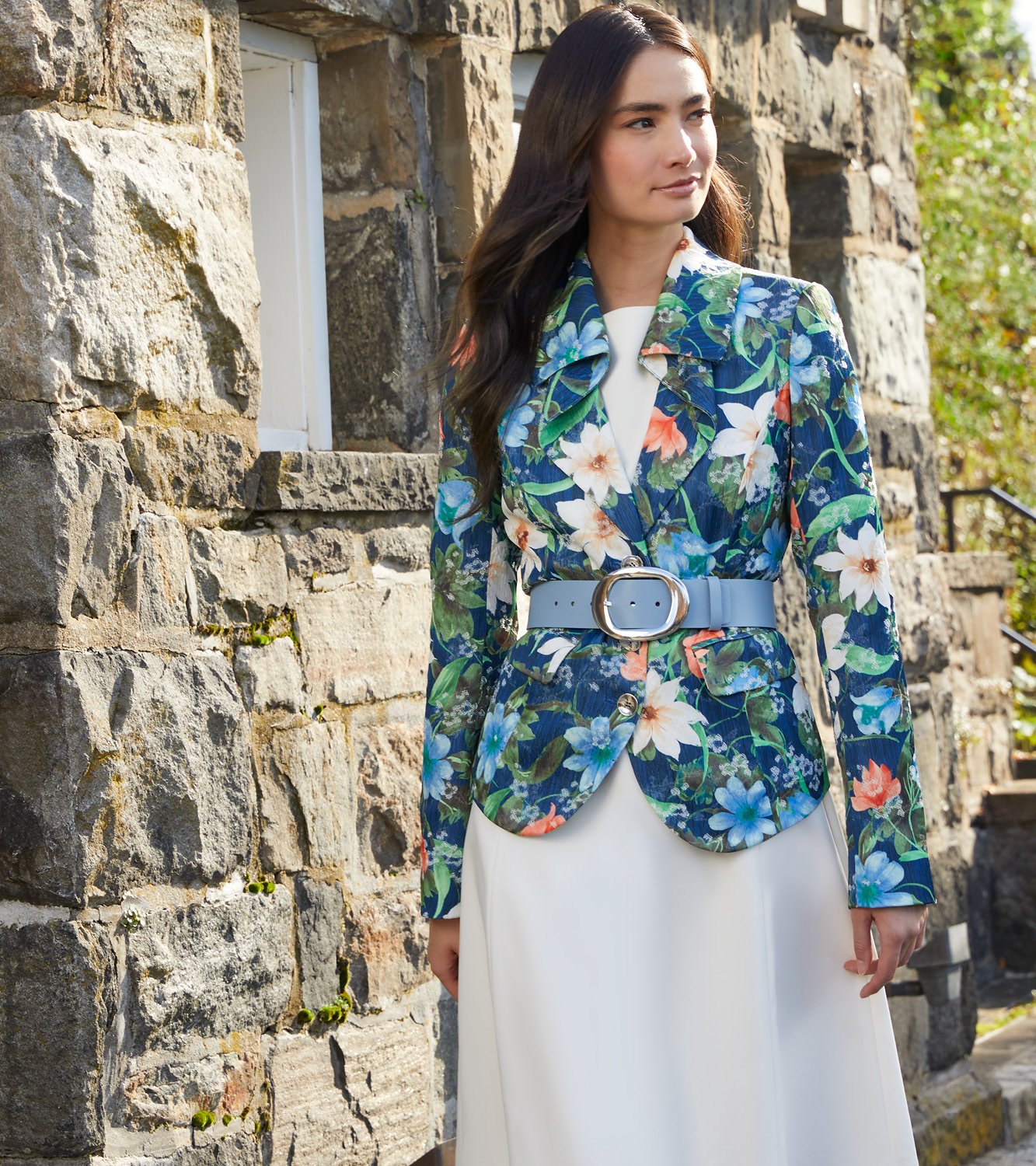In this striking photograph, a woman stands serenely in front of a historic stone building, which features a square window cut out and subtle moss growth accentuating its ancient structure. The bright sunlight bathes the scene, making the vivid colors pop and adding contrast to the image. The woman, with her long hair catching the light to reveal a mix of auburn and brown hues, gazes slightly to the left with a soft, slight smile. Her face is partially illuminated, highlighting her light makeup against her white skin. She is dressed in a vibrant floral print blazer adorned with blue, white, and pink flowers, cinched at the waist by a blue belt with a large silver buckle. Below the blazer, she wears a modest white pleated skirt. The overall composition is both vivid and modest, with the sunlight enhancing the natural and architectural beauty. A glimpse of foliaged branches from a tree adds a touch of nature to the background, complementing the stone building and the woman's colorful attire.